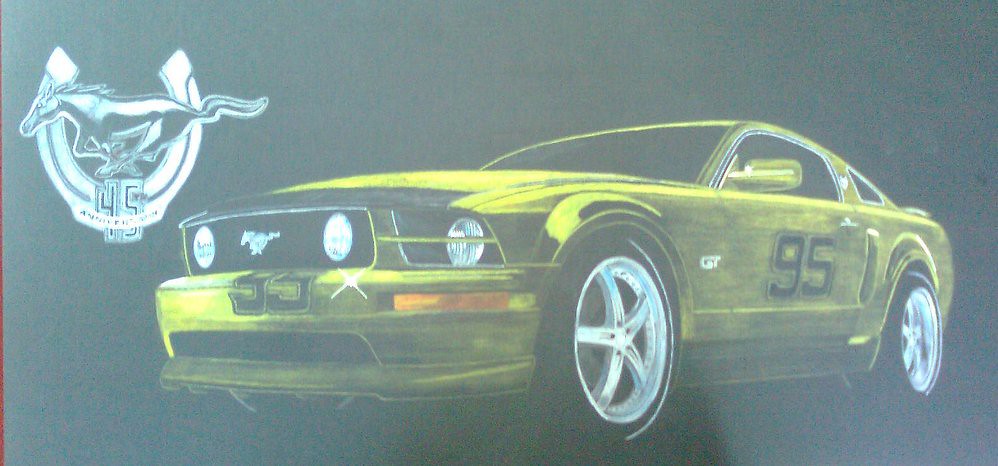The image presents a detailed, somewhat blurry painting of a yellow Ford Mustang muscle car against a black background with a gray-white wash. In the upper left corner, there is a prominent emblem depicting a silver horse in full gallop, encircled by a horseshoe with its bar at the bottom, and the number "45" displayed in black text over the bar. The Mustang, facing forward and slightly to the left, features a bold black "95" on its driver's side door and the Mustang emblem on its black grille. The vehicle is equipped with two round white headlights, additional side lights similar to the front ones, and orange parking lights around the bumper. The front bumper also sports two hooks. The car's tires boast black rims with silver five-star hubcaps, and the windows are tinted black.